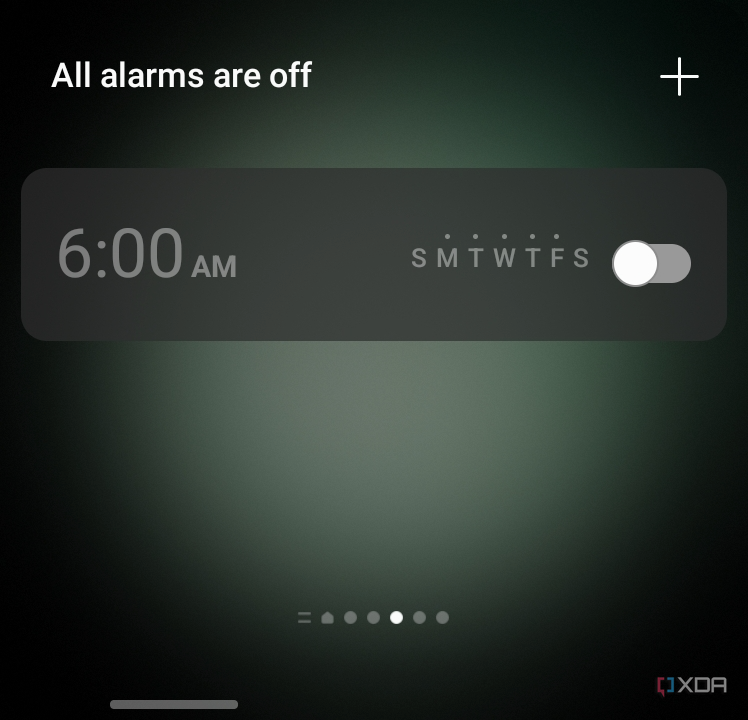This image depicts a screenshot of a digital device, showcasing a minimalist design with a gradient background transitioning from black to gray. The gradient is darker around the outer edges, drawing focus inward. The image itself is square-shaped.

In the top-left corner, text in white reads, "All alarms are off." On the top-right corner, there is a small plus sign, likely indicating the option to add a new alarm. Below this corner is an alarm time display set for "6 a.m." This time is enclosed in a dark gray rounded rectangle. Adjacent to the time display are the letters "SMTWTFS," indicating the days of the week, each with a dot centered above their respective initials. The highlighted days—Monday, Tuesday, Wednesday, Thursday, and Friday—signify when the alarm is set to go off, although the toggle switch beside this section is currently turned off, confirming that the alarm is not active.

Below this central information display, a series of navigation dots appear, with the middle dot highlighted in white to show the current page of the interface. Additional navigational elements include two lines at the start and a home button among the five dots. 

At the bottom of the screen, a lighter gray rounded rectangle houses more features, with the rightmost section displaying "XDR" along with a small icon featuring a red and green outlined box, potentially a status indicator or a different function symbol.

This detailed layout effectively communicates the device's alarm settings and navigational structure using a clean, intuitive interface.